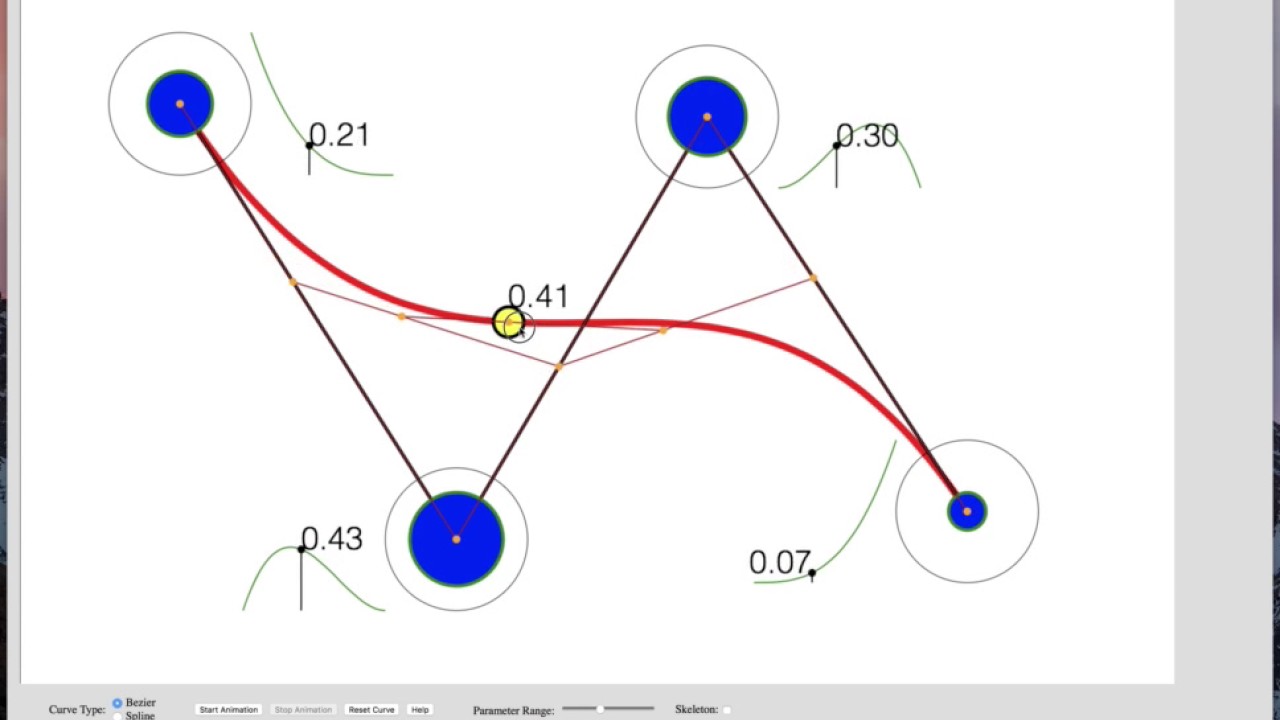The image displays a detailed diagram, possibly from a graphics program, featuring four blue circles of varying sizes connected by black lines in a zigzag pattern. Each circle is encircled by a larger black outline and contains a small yellow dot. The circles are positioned on a white background with associated numerical labels: 0.21 in the upper left, 0.43 in the lower middle, 0.30 in the upper middle, and 0.07 in the lower right. These connections and points are further illustrated by a wavy red line that snakes its way from the bottom right to the top left, weaving through each blue circle. Near the bottom of the diagram, barely legible text details options typical of a graphics program interface, such as curve type selection (Bezier or spline), and buttons for starting, stopping, or resetting an animation. The presence of a parameter range slider and a skeleton checkbox suggests this diagram is meant to demonstrate the construction of a Bezier curve.